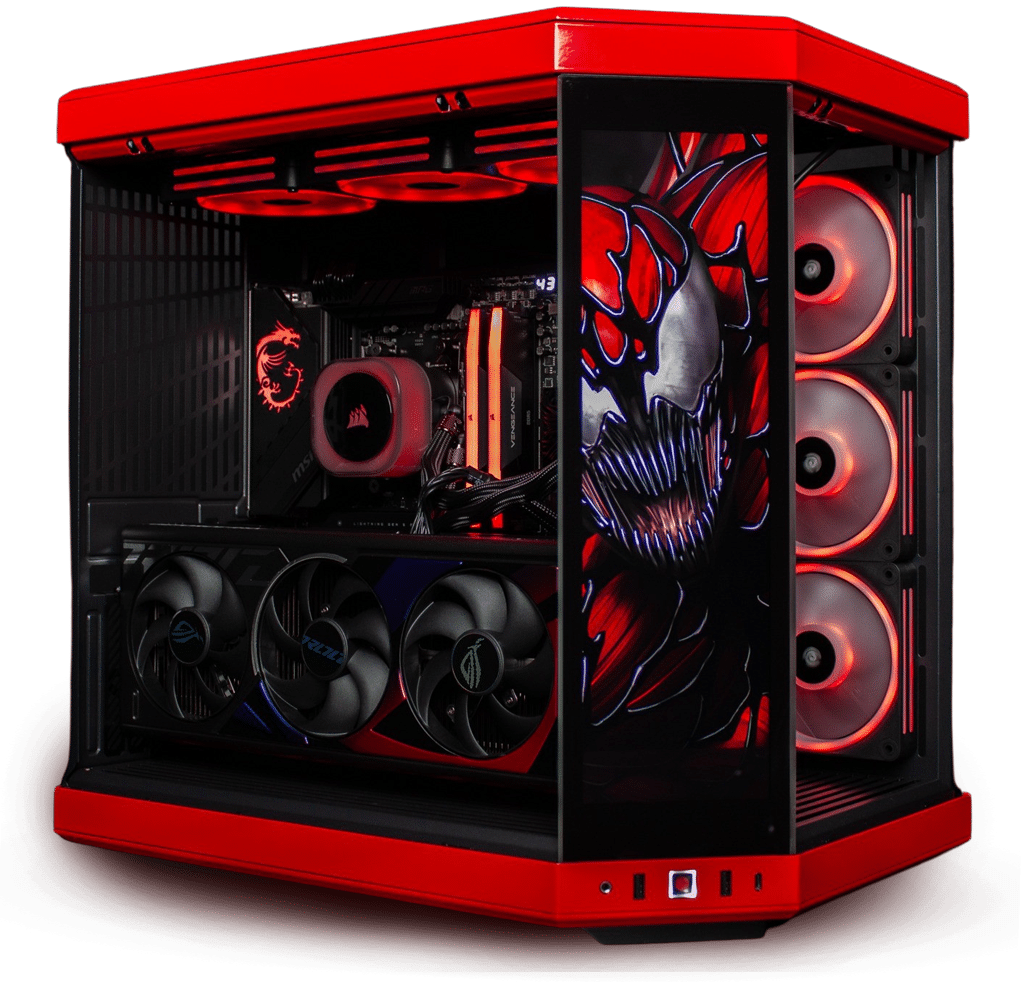This image displays a high-end desktop gaming computer set against a solid white background. The computer case is a striking, bright red with transparent panels, allowing a clear view of the internal components. Neon lights illuminate the inside, highlighting the three large fans and various electrical components, including the CPU and motherboard, which is designed to resemble a work of art. The case features a tall rectangular side panel adorned with a dramatic graphic of a dark, villainous figure resembling Venom from Spider-Man, characterized by its cat-shaped gray eyes and long, menacing metal teeth. Despite its sleek and tech-laden appearance, the overall color scheme is dominated by red and black. Additionally, the front panel includes practical elements such as a microphone jack and several USB ports, making the setup as functional as it is visually striking.